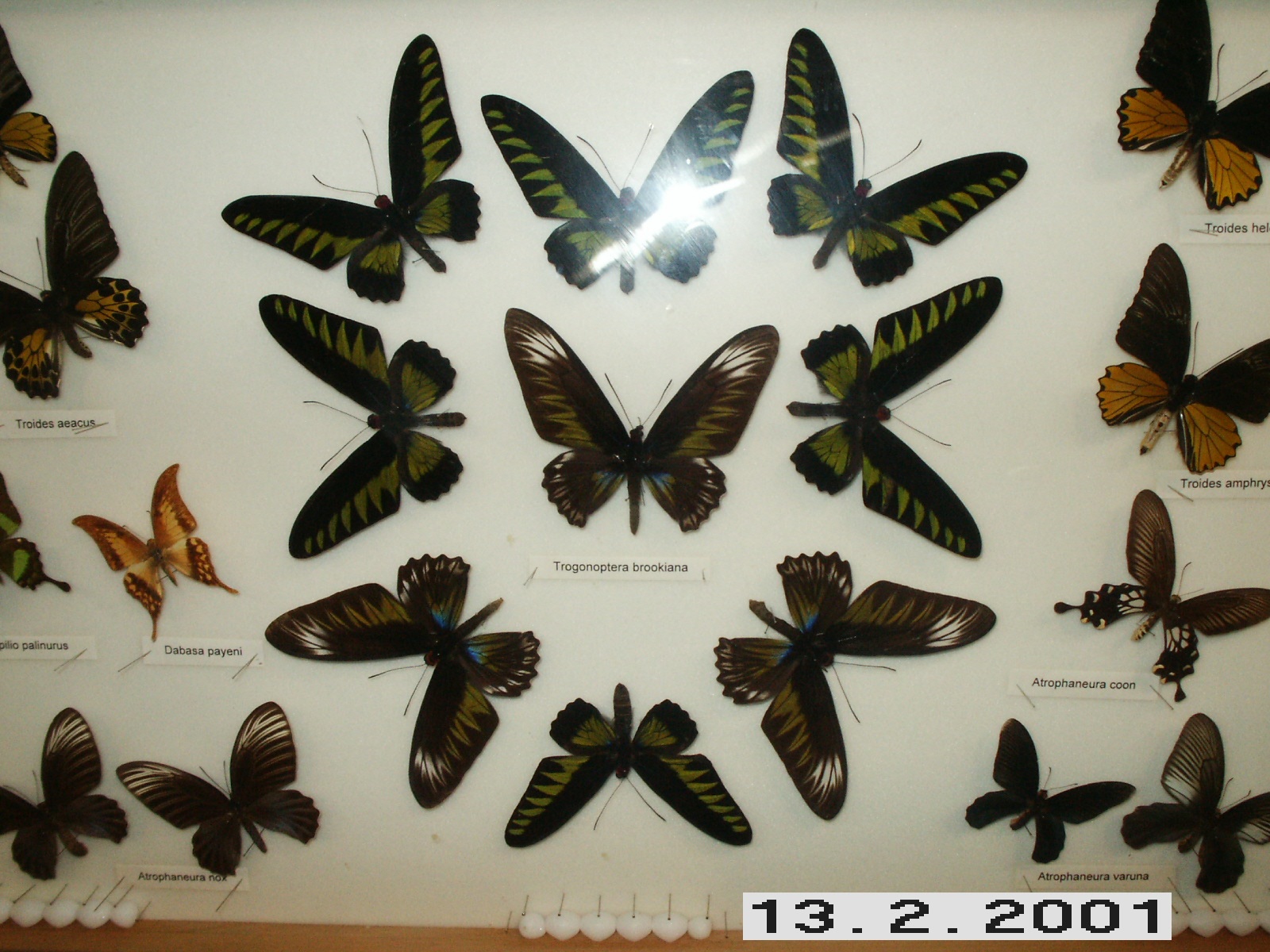This indoor, full-color photograph showcases an intricately arranged butterfly collection behind a glass or plastic case, with notable reflections, including a camera flash in the upper center of the image. Set against a white background, the butterflies are organized into a detailed and symmetrical pattern. On either side, butterflies are aligned diagonally from the bottom corners, moving towards the top corners. The left and right sides each feature two rows of butterflies in various colors, including green and black, brown and yellow, and yellow and black, with pairs of each species positioned next to one another. At the center of this formation is a circle of butterflies surrounding a central specimen, all of the same species, identified as Trogonoptera brooklana by a label beneath it. Each butterfly is accompanied by a small tag displaying its name in black font, pinned next to it. A subtle date indicating February 13th, 2001, is visible in the lower right corner of the image.